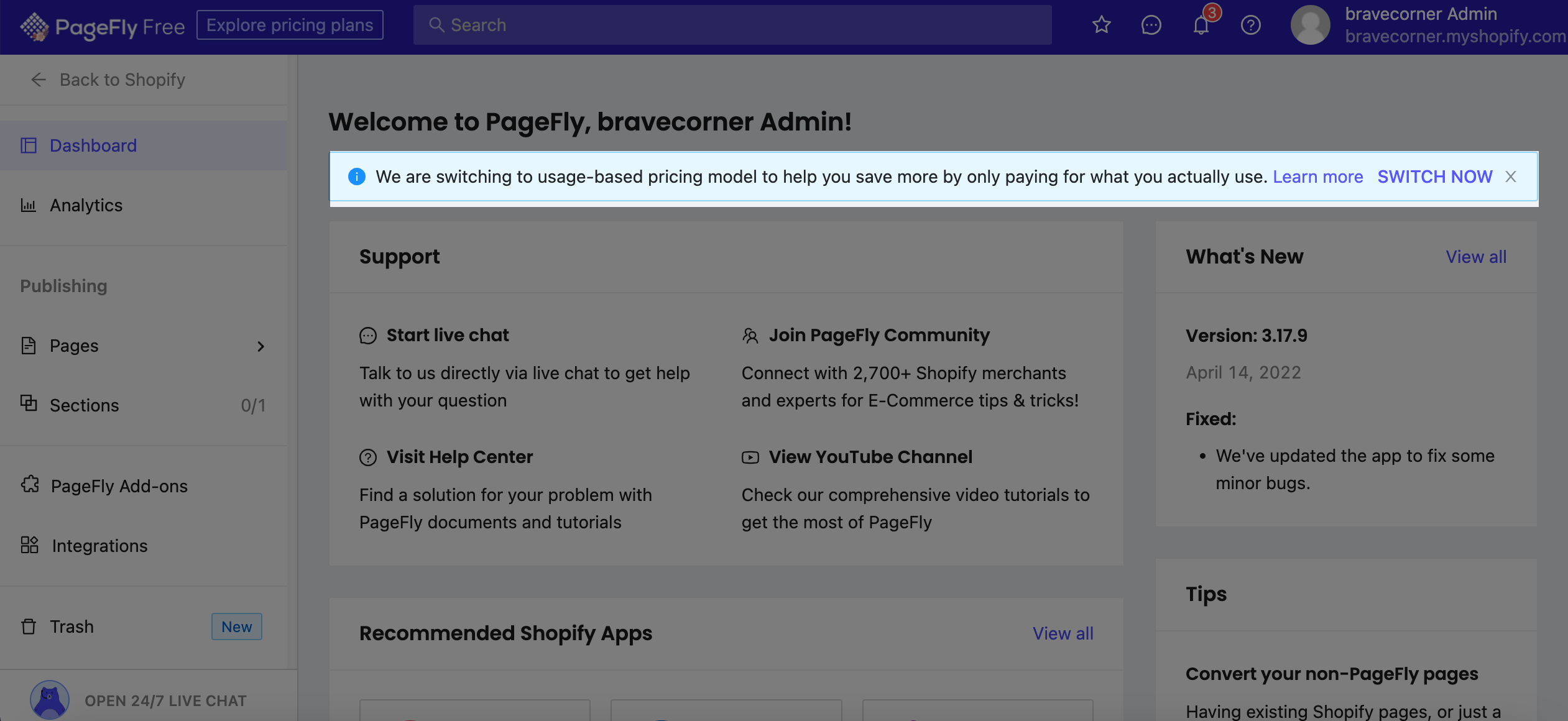Screenshot Description: PageFly Interface on Shopify

The screenshot displays the PageFly application interface integrated with Shopify. The application interface features a prominent blue banner at the top, extending across the entire width of the screen. On the left side of this blue banner, there is a white icon resembling a chessboard viewed diagonally. Adjacent to this icon, there is a three-part label: "PageFly Free." Here, "Page" and "Fly" are capitalized and merged into one word, while "Free" follows it.

To the right of this label, there is a button labeled "Explore Pricing Plans." At the far right end of the banner, user information is displayed as "Brave Corner Admin" followed by the URL "bravecorner.myshopify.com," indicating that this tool is indeed used with Shopify.

Beneath the blue banner, on the left side, there is a vertical column of submenu options on a gray background. This column starts right under the PageFly icon and includes the following menu items:
- A "Back to Shopify" option with a left-pointing arrow.
- "Dashboard" (highlighted).
- "Analytics."
- "Publishing."
- "Pages" (with a right-pointing arrow indicating submenus).
- "Sections."
- "PageFly Add-ons."
- "Integrations."
- "Trash."

The main section of the screen, making up about three-quarters of the interface's width, is dedicated to the content area. This section is headed by a welcome message that reads "Welcome to PageFly Brave Corner Admin." Overlaid on this message is a white pop-up button stating, "We’re switching to a usage-based pricing model to help you save more by only paying for what you actually use. Learn more and switch now," suggesting it is clickable.

Below this pop-up, there is a support section offering four options:
- "Start Live Chat."
- "Visit Help Center."
- "Join PageFly Community."
- "View YouTube Channel."

To the right of these options, a lighter gray text box highlights what's new in version 3.17.9 (dated April 14th, 2022), including a note about minor bug fixes.

The bottom part of this content area mentions "Recommended Shopify Apps," though the text is partially cut off, and another recommendation titled "Tips: Convert your non-PageFly pages."

This comprehensive layout indicates a well-organized interface designed to assist users in navigating the PageFly application within a Shopify environment efficiently.